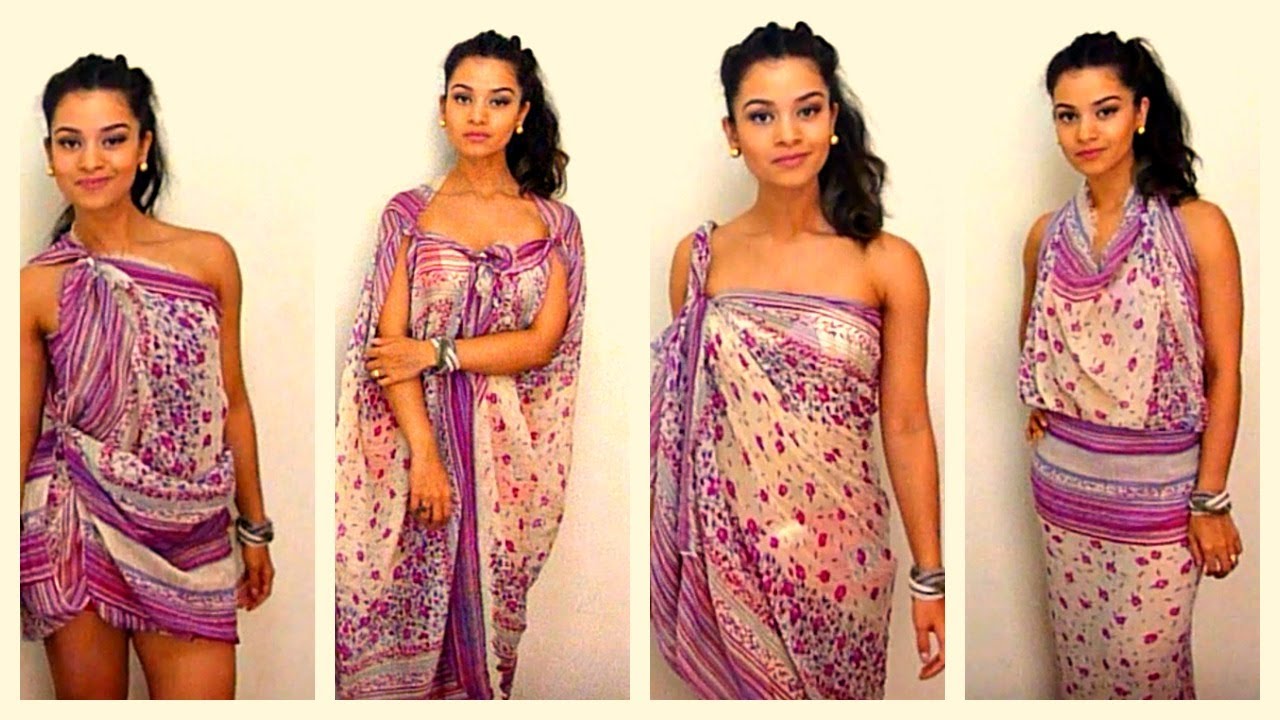The image showcases a collage of an elegant woman, presumably an Indian model, demonstrating various stylish ways to wrap a scarf into different outfits. The collage consists of four pictures, each bordered by thin white lines and set against a consistent pink background. 

In every image, the woman retains a graceful demeanor with her long black hair tied back in a messy ponytail and accessorized with a wristband and earrings. She is dressed in a scarf featuring a cream background adorned with pink floral patterns and purple lines.

In the first picture, she wears the scarf as a chic, asymmetrical mini-dress, draped over one shoulder and tied at the waist, creating a look that ends just above her knees. She stands confidently, smiling.

In the second picture, the scarf transforms into a cover-up with a sporty yet elegant vibe. It is tied over both shoulders and cinched at the center, forming a front opening that runs down her body. One of her arms is bent at the elbow, while the other hangs naturally by her side.

In the third photo, the scarf is styled as a longer dress, again draped over one shoulder but this time extending below her knees. Her arms are relaxed at her sides, showcasing the elongating effect of the outfit.

In the final picture, the scarf is fashioned into a form-fitting long skirt with a looser, halter-style top. The scarf is tied behind her neck, and she poses sideways with one hand on her hip and the other by her side.

Together, these images artfully present the versatility and beauty of the scarf when transformed into various fashionable attire.